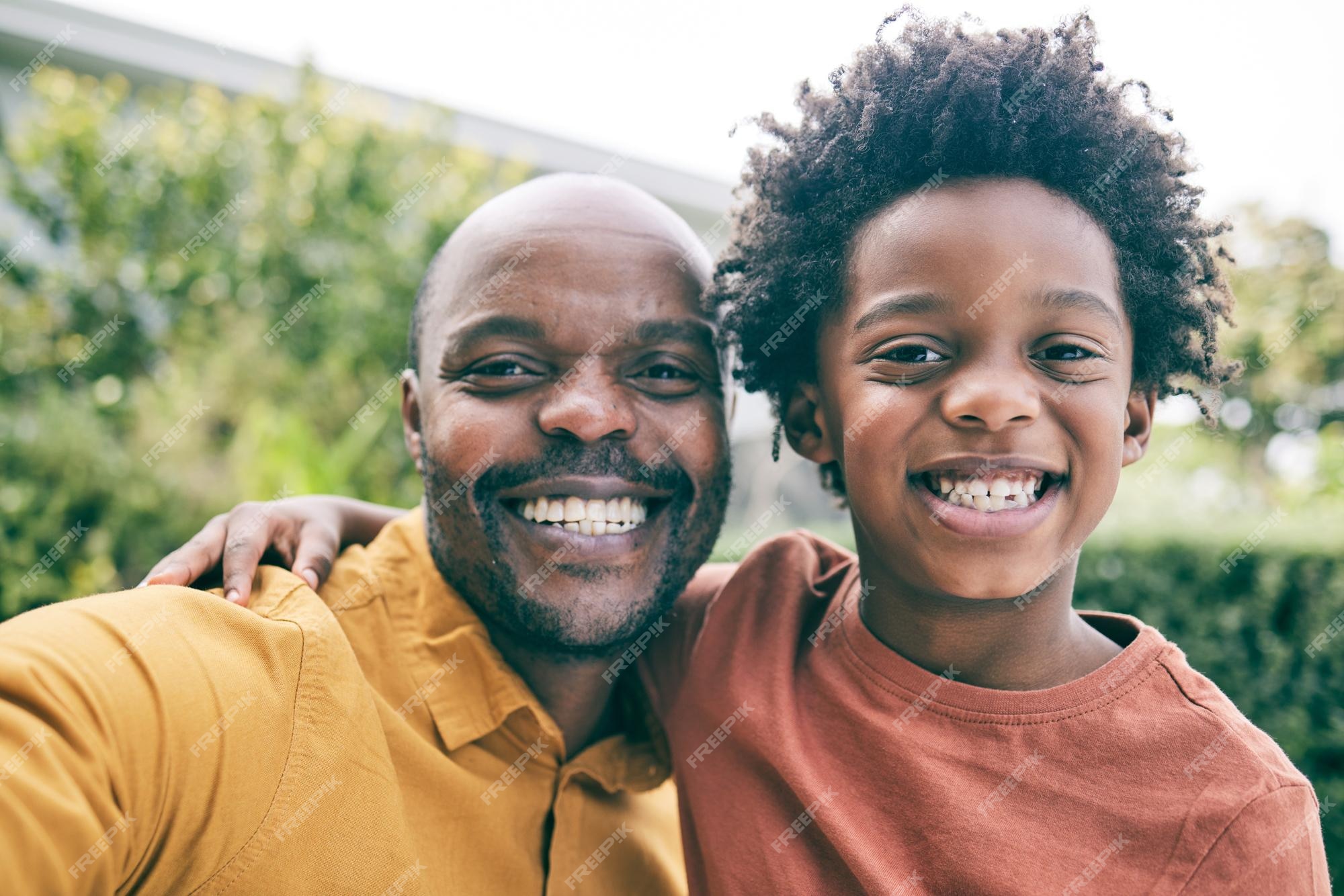In this close-up selfie, an African-American father and son are captured outdoors, surrounded by lush greenery with bushes and trees visible in the background, and a light yellow sky suggesting it's either dawn or dusk. Positioned on the left, the father, around 40 years old, sports a bald head along with a bit of a beard and wears a bright yellow collared, long-sleeve dress shirt. On the right, his son, approximately 10 years old, has fluffy, curly hair reminiscent of an afro and is dressed in a vivid red shirt. Both are smiling broadly, showing their teeth, radiating joy and warmth. The image is marked with a 'Freepik' watermark, rotated 45 degrees counterclockwise and scattered across the picture, indicating its usage rights.